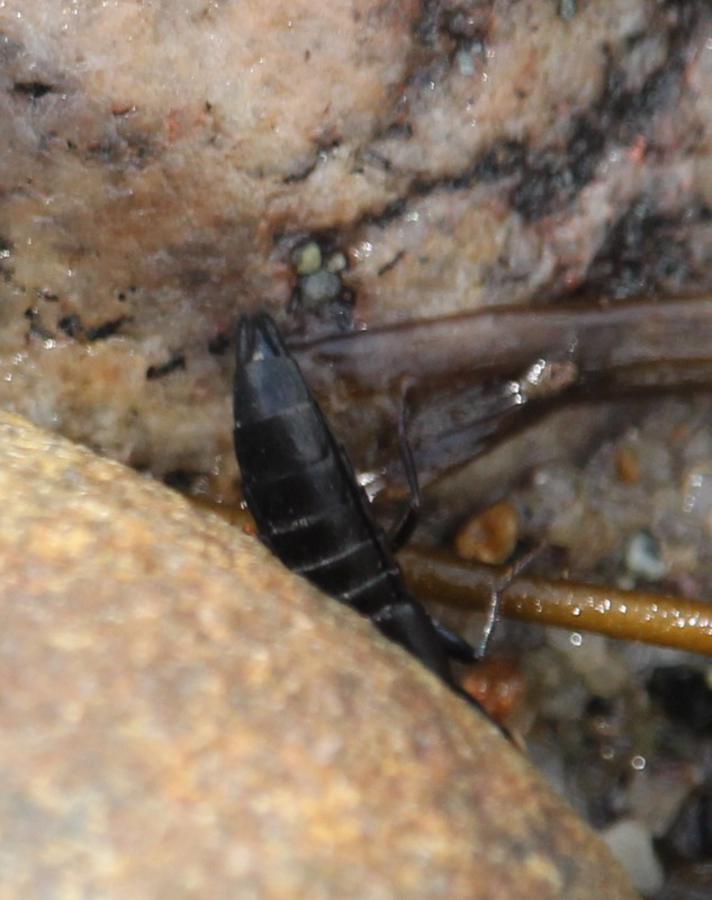This image is an extreme close-up of a black insect nestled within a rocky surface. The central focus is the segmented black body of the insect, which appears to be upside down. You can discern a leg extending from the bottom right side of its body, contributing to the insect-like appearance. Surrounding the insect is a rocky environment with a granite-like texture; light in color with dark splotches and crevices throughout it. On the right side of the photograph, there's an orange rod-like structure which could be a stick or branch. The overall setting seems to be either underwater or among rocks, and while initially ambiguous, a closer look aligns more with the idea of an insect amid a rocky crevice rather than seaweed.